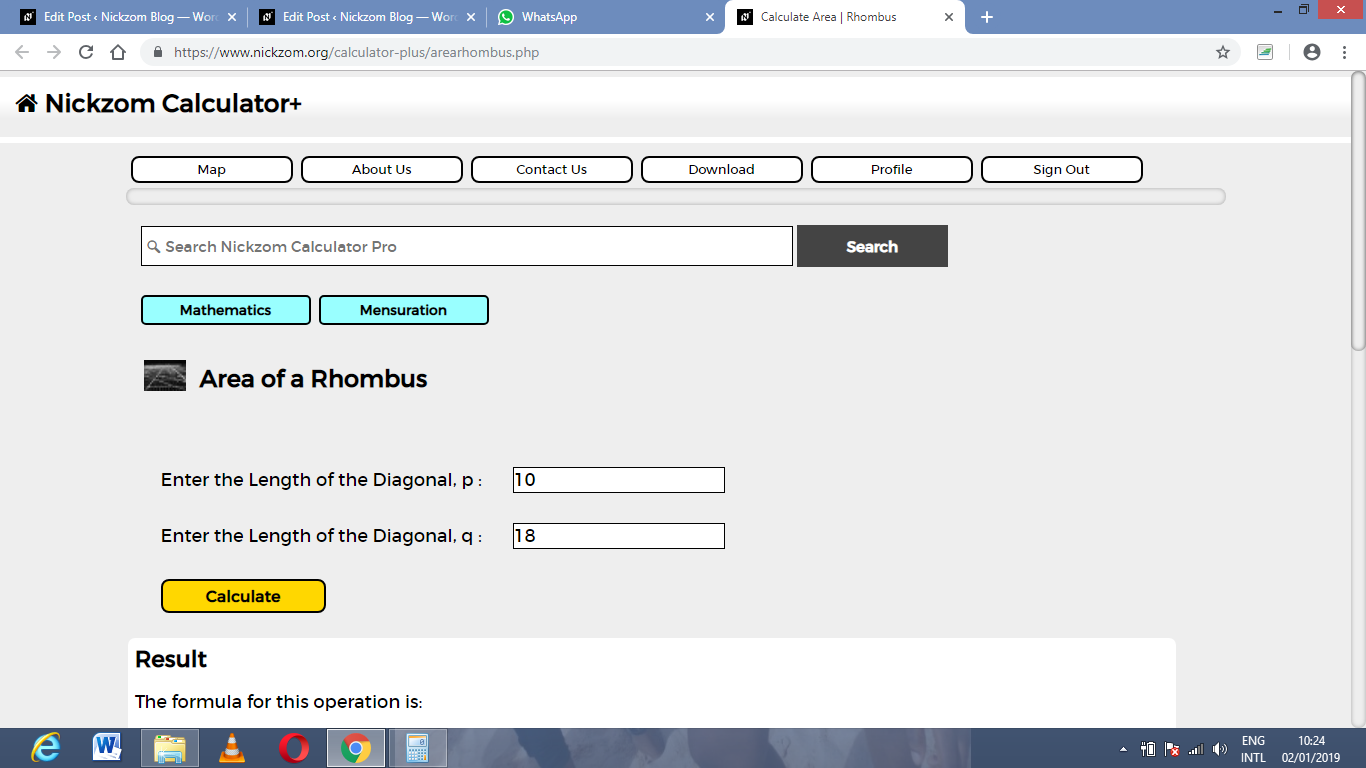The image depicts a computer browser with multiple tabs open. The tabs are labeled "Edit Post," "Edit Post," "WhatsApp," and the currently active tab titled "Calculate Area Rhombus." The visible portion of the browser displays the website "Nik Zom Calculator Plus." 

At the top of the page, there are navigation options including "Map," "About Us," "Contact Us," "Download," "Profile," and "Sign Out." Below these options is a search bar labeled "Search Nik Zom Calculator Pro," with a search button on its right.

Further down the page, there are two rectangular buttons labeled "Mathematics" and "Menstruation." Below these buttons, the heading "Area of Rhombus" is prominently displayed. The user is prompted to input values for the length of the diagonals with instructions stating, "Enter the length of the diagonal, P," with an input number of 10, and "Enter the length of the diagonal, Q," with an input number of 18. A button labeled "Calculate Rhombus" is situated beneath these inputs. Below this button, there is a section labeled "Result" followed by an explanation of the formula for the operation.

At the bottom of the screen, a taskbar displays various application icons including Internet Explorer, Microsoft Word, a document folder, files, a media player cone icon, a red "O" icon, Google Chrome, and a calculator.